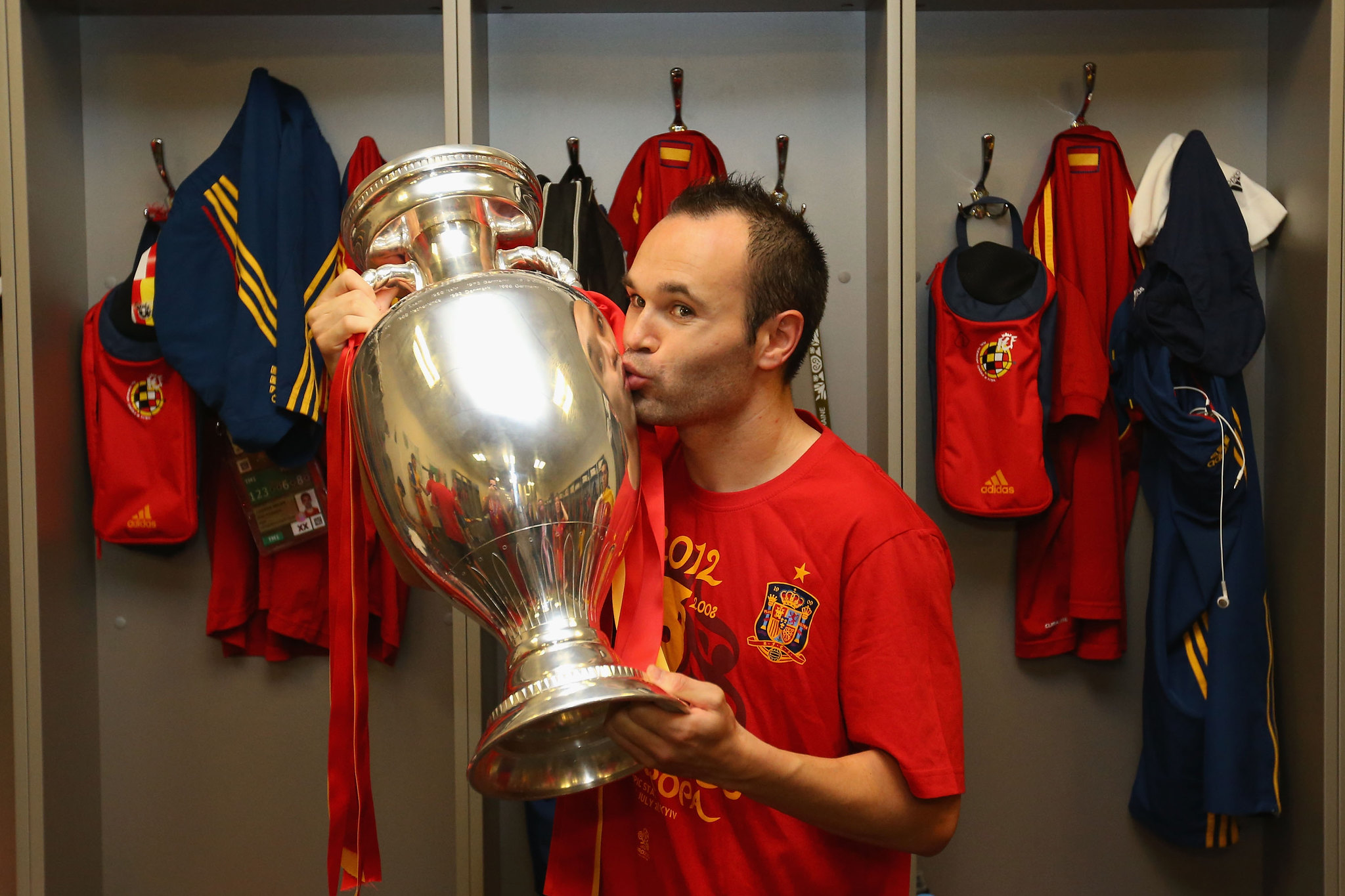In the center of this indoor image, an athlete proudly kisses a shiny, reflective silver trophy, clearly in the midst of a celebration. He is dressed in a red shirt, likely celebrating a championship, with distinctive yellowish-orange text and stripes, indicative of a soccer (football) team. Surrounding him in the background are blue lockers adorned with yellow stripes, filled with an assortment of team gear and athletic apparel, including several bags and varied clothing items. The scene suggests it is set in a locker room, given the abundance of sports-related gear and specific blue-and-yellow decor. The athlete, possibly affiliated with Barcelona as suggested by the numerous Barcelona-themed items, stands directly at the center of the image, creating a vivid focal point of triumph against the cluttered backdrop of athletic storage and gear.